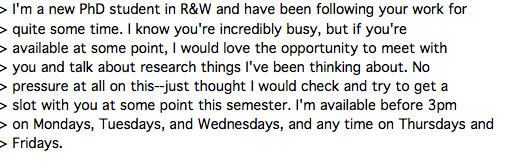The image displays a small, rectangular white box filled entirely with black text against the white background. The text appears centered and consists of a detailed message resembling a reply in an email chain, as indicated by the right-facing carets at the beginning of each line. The message reads: "I'm a new PhD student in R&W and have been following your work for quite some time. I know you're incredibly busy, but if you're available at some point, I would love the opportunity to meet with you and talk about research things I've been thinking about. No pressure at all on this—just thought I would check and try to get a slot with you at some point this semester. I'm available before 3 p.m. on Mondays, Tuesdays, and Wednesdays, and anytime on Thursdays and Fridays." This monochromatic image emphasizes the simplicity and formality of the communication, likely a professional request for a meeting.